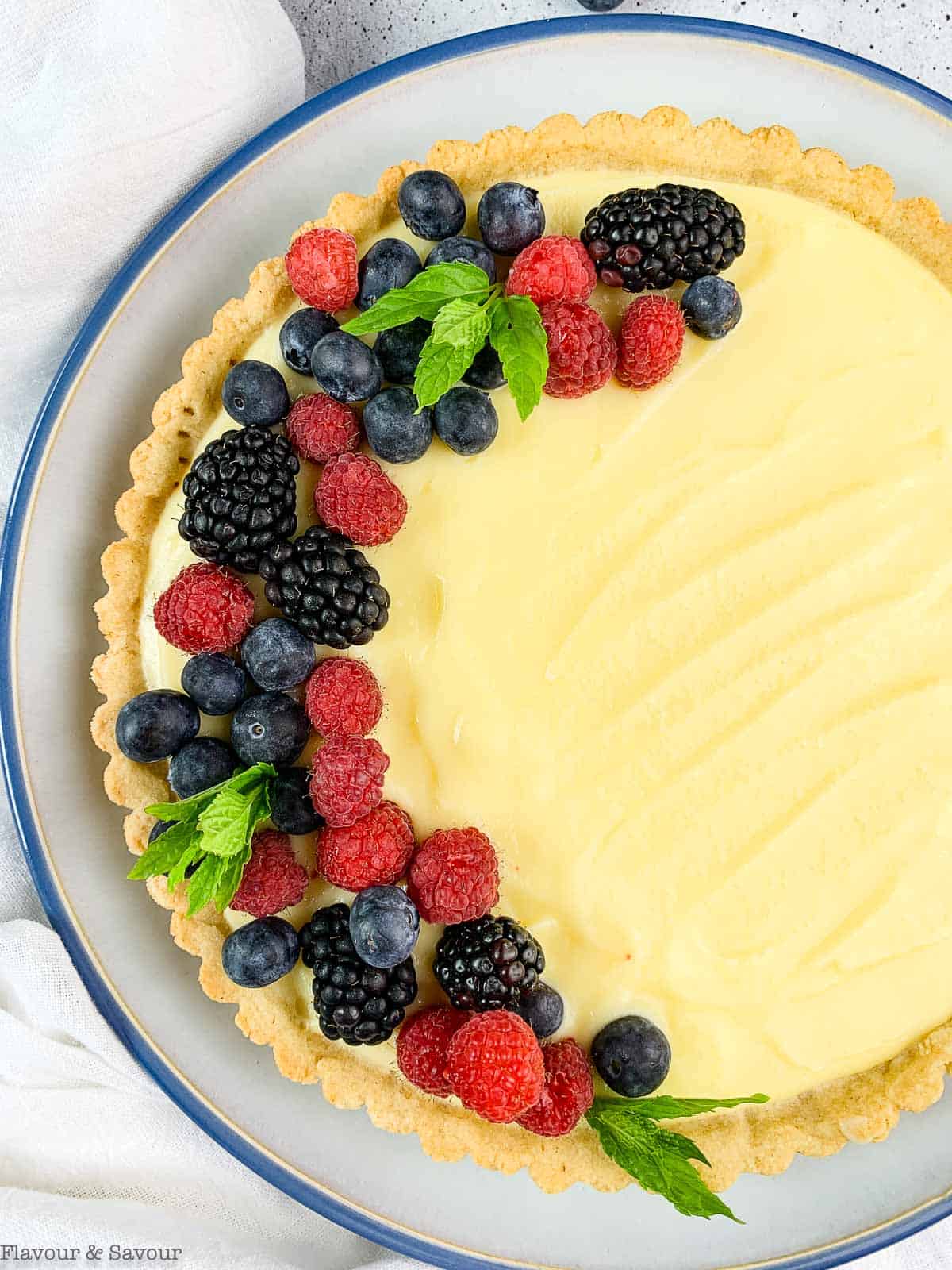The image features a beautifully presented pie, which gives the impression of being freshly made. It rests on a white, speckled table, possibly a marble countertop. The pie is set on a round white plate with a blue trim, and nearby, a white napkin or fabric is folded. The bottom left-hand corner of the image has the words "Flavor and Savor" in black letters. The pie itself has a light brown, graham cracker-like crust and a smooth, yellow frosted surface, where knife marks are faintly visible. The left half of the pie is artfully adorned with a variety of fresh berries, including blueberries, raspberries, blackberries, and boysenberries, along with a few green mint leaves. This vibrant, berry-topped crescent contrasts with the plain right half of the pie, creating a visually appealing presentation.